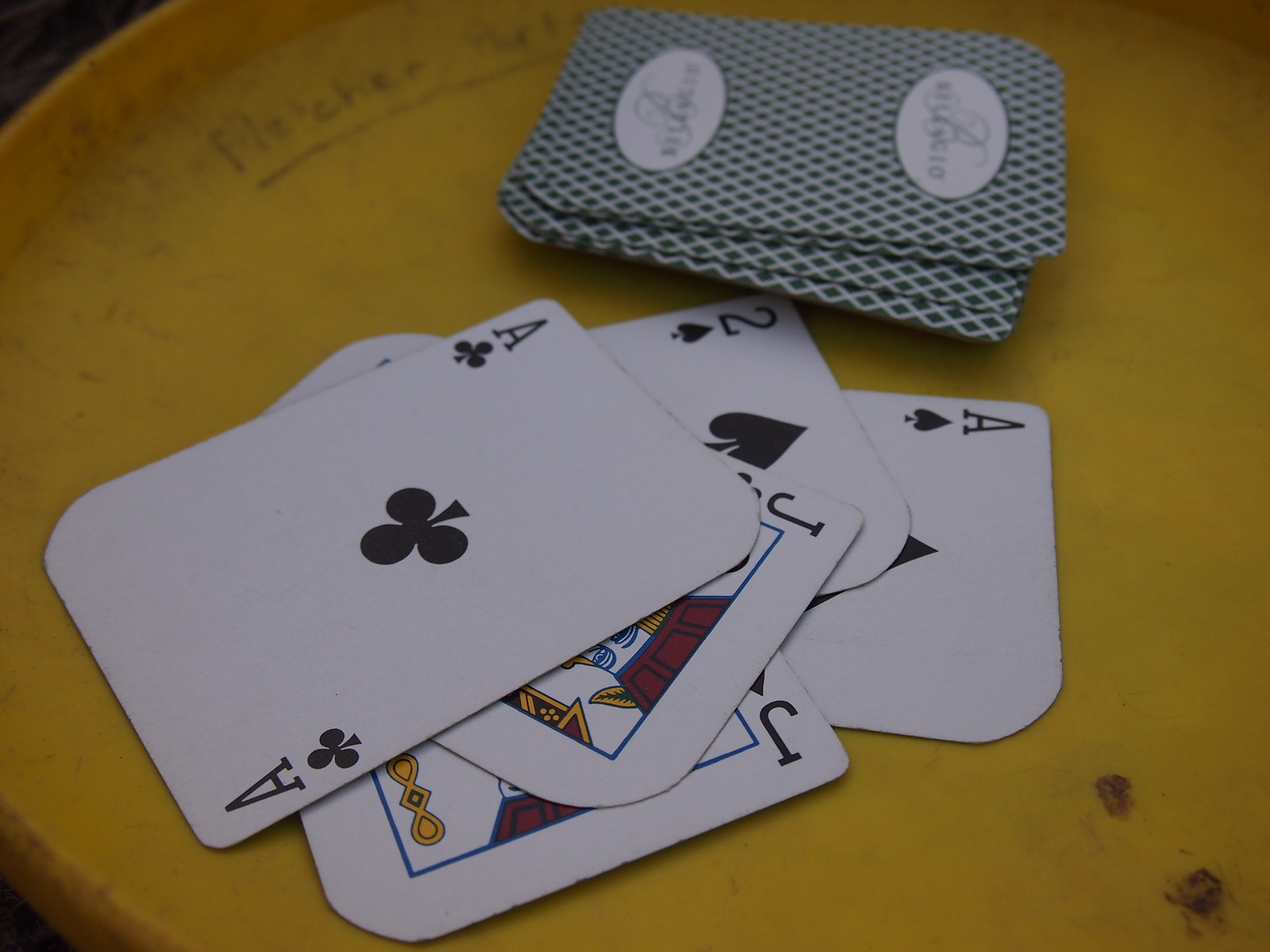A scattered pile of playing cards lies atop a distressed, light wood table, the surface marked by the etched word "Fletcher," likely scratched in with a pencil. Five cards are clearly visible: the Ace of Spades, the Ace of Clubs, the Two of Spades, the Jack of Clubs, and the Jack of Spades, forming a strong two-pair poker hand. The backs of the cards feature an intricate design, adorned with a prominent, ornate letter 'B,' though it's difficult to discern finer details due to the blur. The scene is bathed in dim lighting, with the photograph's edges softly out of focus, enhancing the antique and quaint atmosphere of the setting.